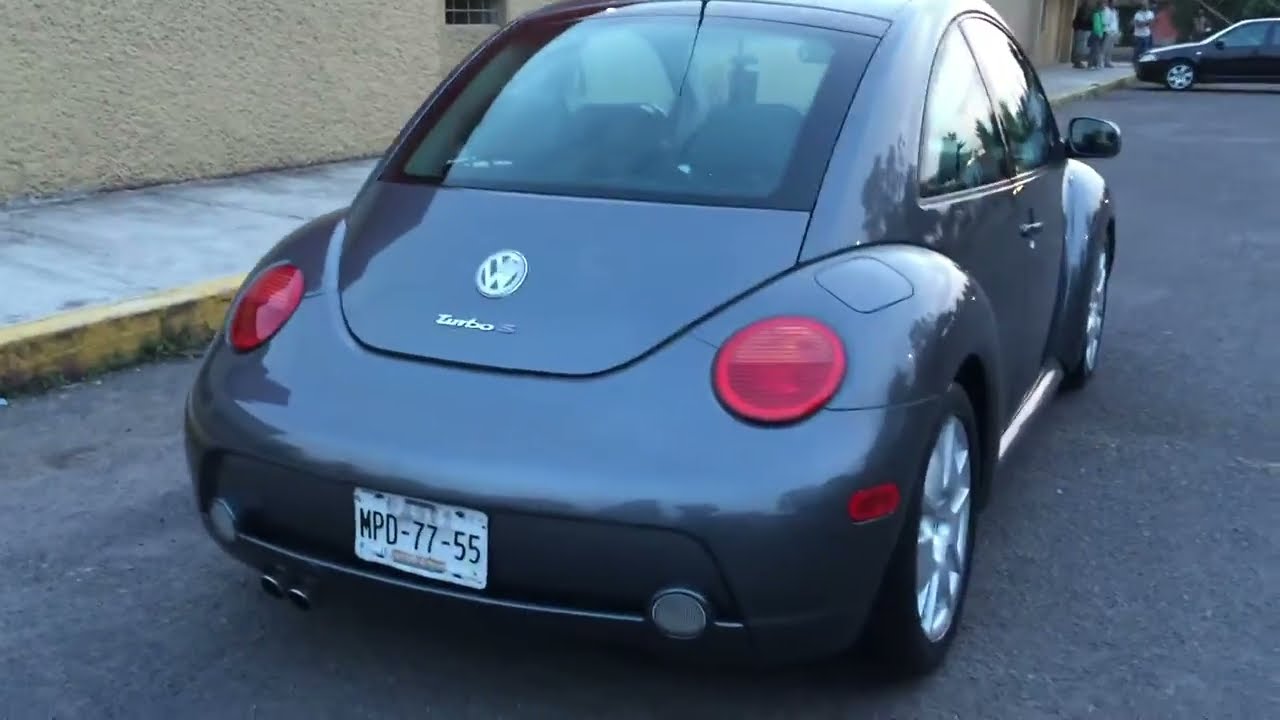The photograph captures the back end of a dark gray or black modern Volkswagen Beetle parked on a gray concrete street next to a yellow-bordered sidewalk. The image is a close-up, showing the iconic VW logo and the word "Turbo" beneath it, along with the license plate reading "MPD-77-55." Twin muffler pipes are visible on the left side beneath the car. The rear lights are red, and you can distinctly see the back windshield and the right-side mirror, as the car is angled slightly to the left. In the background to the upper left, there is a building with a stucco or concrete surface, featuring a window with bars. To the upper right, another black car is partially visible with a few people standing in front, milling about on the sidewalk.